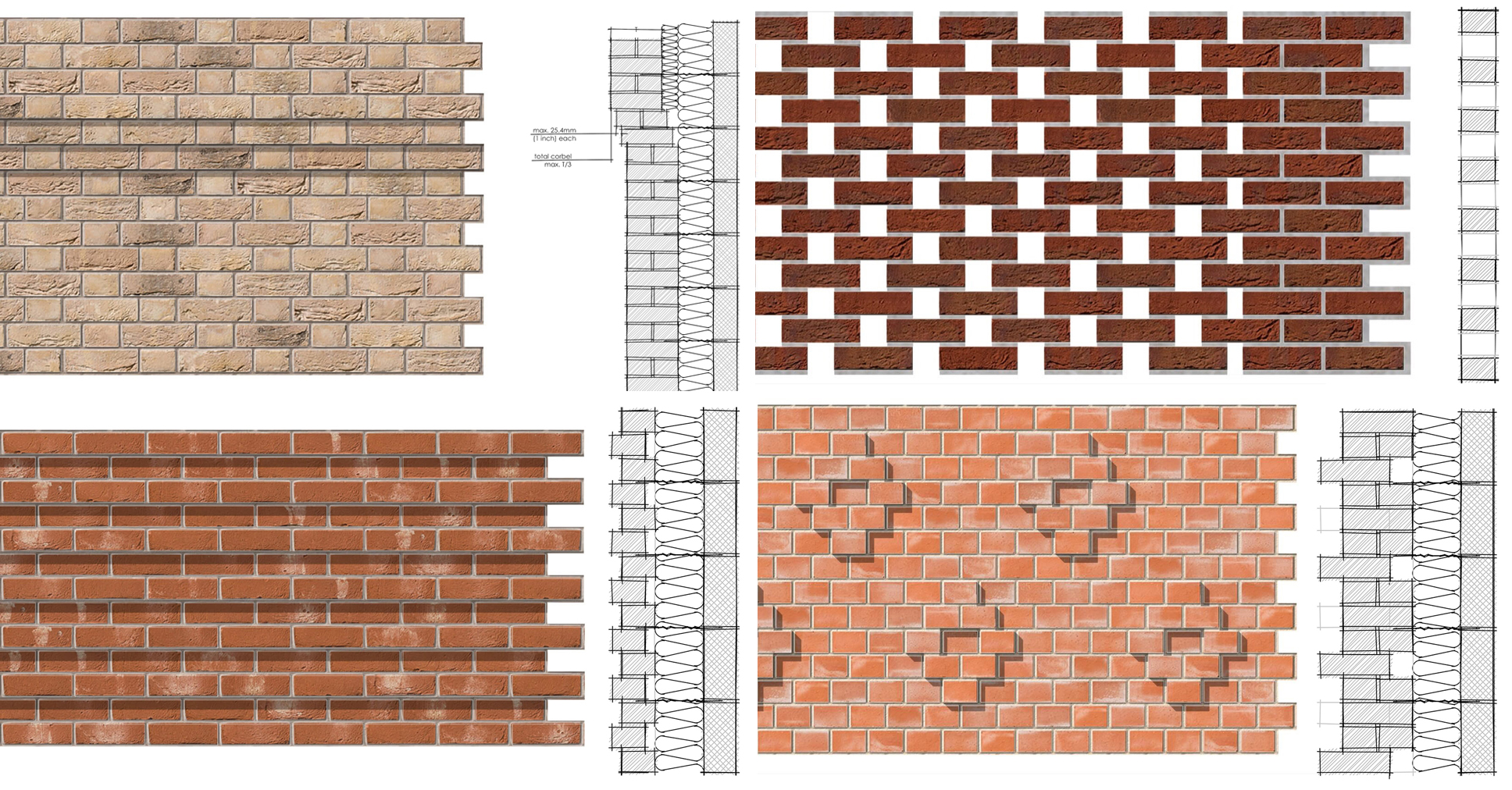This image, seemingly created for an exterior design website, is a detailed collage showcasing four distinct brick masonry patterns and colors, arranged in two rows with two sections each. Each section presents the face of the brick wall alongside a side profile diagram that illustrates how the bricks are arranged in a three-dimensional perspective. 

In the top left, there is a light tan brick pattern, with variations in shades of tan and a relatively uniform surface with fewer bricks jutting out. To the right of this section, there is a darker brownish-red brick pattern with noticeable wide gaps between the bricks, making some bricks appear missing.

At the bottom left, a traditional red brick pattern features rows where every other row is indented, creating a staggered effect. On the bottom right, a terracotta red pattern shows shorter bricks with intricate diamond-shaped designs on the surface, giving a textured, decorative look. 

The side profiles beside each of these sections provide an additional perspective, showing how the bricks either pop out or remain indented, adding to the overall visual diversity of the masonry designs.